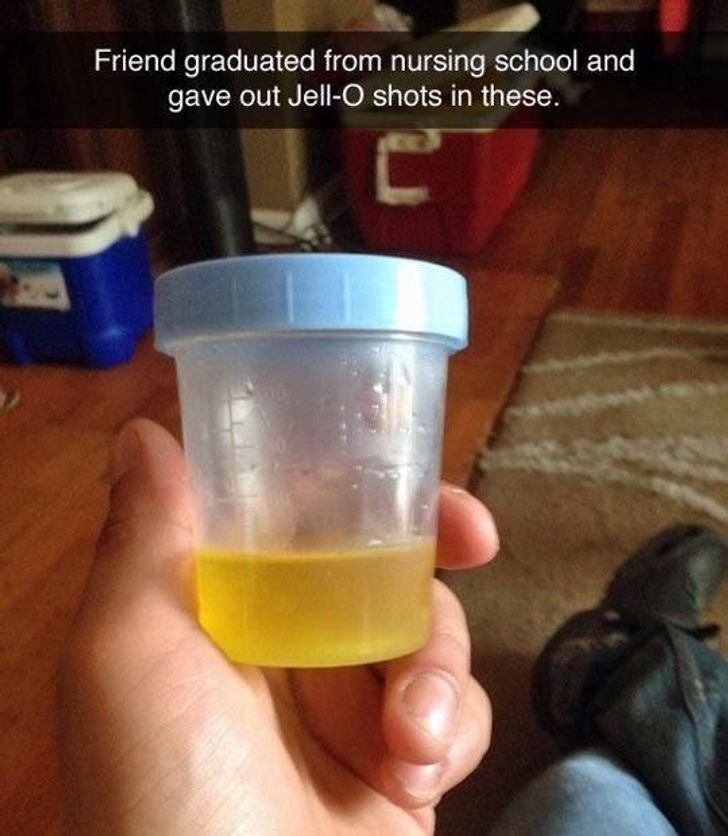In this photo, a Caucasian male is holding a closed, translucent plastic specimen cup commonly used for urine samples. The cup contains a small amount of yellow liquid, likely yellow jello, mimicking the appearance of urine. The image includes a humorous caption at the top that reads, "Friend graduated from nursing school and gave out jello shots in these." The person's hand is visible, along with part of their knee clad in blue jeans and black leather boots. The setting appears to be a room with a wooden floor, featuring red and blue coolers, a brown rug with white stripes, resembling a vine pattern, and hints of a casual or possibly party atmosphere.